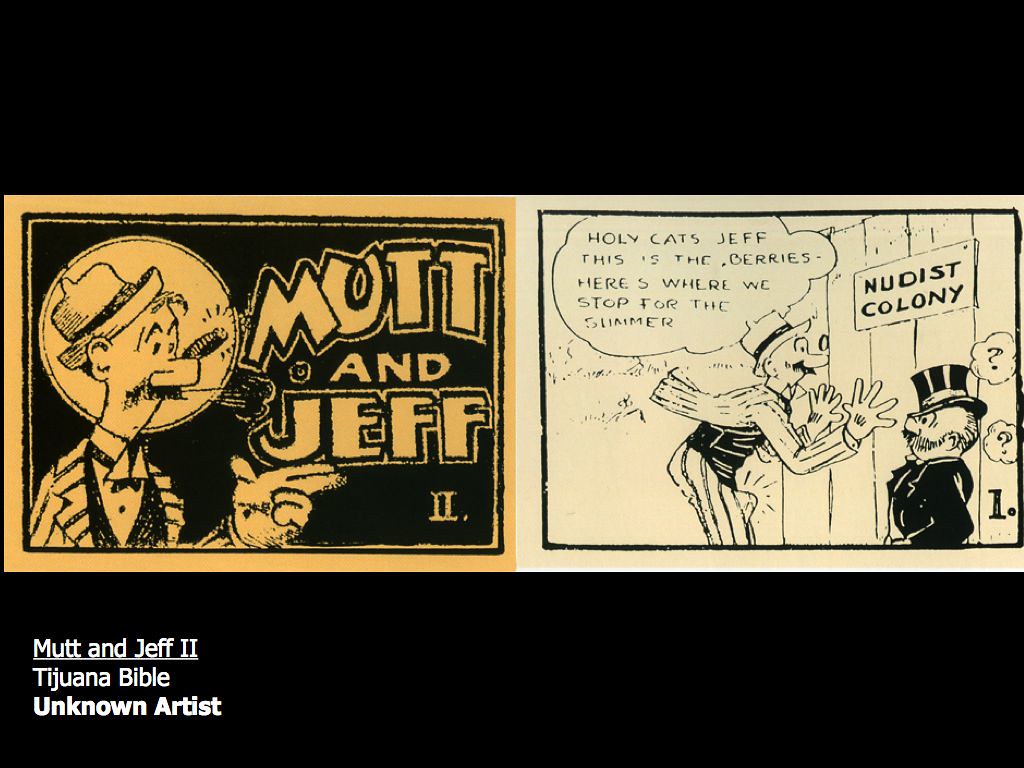The image features a comic strip set against a black background, spotlighting the classic cartoon characters Mutt and Jeff. On the left side, the panel displays a gold and black logo reading "Mutt and Jeff II," alongside an image of a man in a hat, with a cigar, a mustache, a bow tie, and a goofy-looking suit. This character is pointing to the right. The right side of the panel reveals the actual comic strip. In this scene, Mutt peeks through a hole in a wooden fence marked by a sign that reads "Nudist Colony." He exclaims, "Holy cats Jeff, this is the berries. Here's where we stop for the summer." Jeff, a small man with long sideburns, a top hat, and a black suit, appears confused, with question mark bubbles indicating his bewilderment. Adding to the contextual details, the strip is labeled at the bottom with "Mutt and Jeff II, Tijuana Bible, unknown artist." This suggests that the piece may be part of a series, specifically a Tijuana Bible, which is an underground comic from an unknown artist.